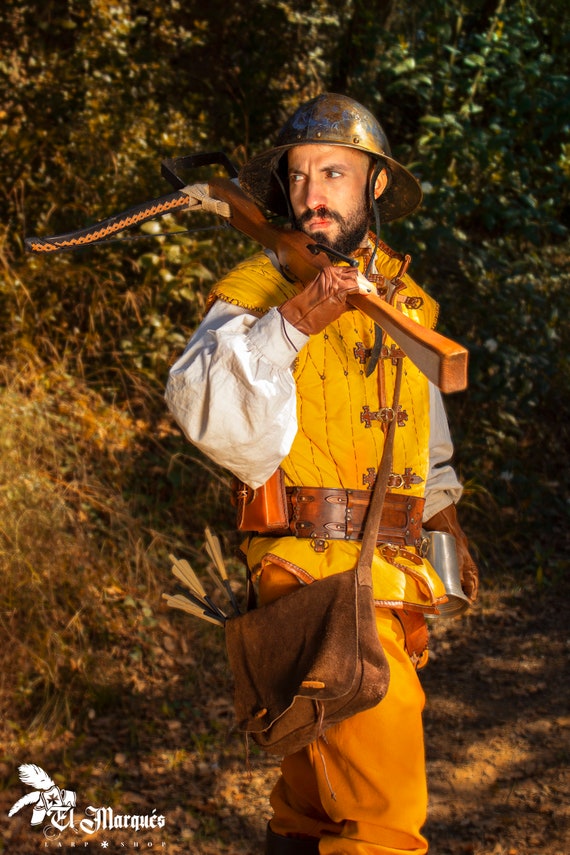This color portrait photograph features a man in his 30s dressed as a medieval soldier, standing in a forest setting with hints of leaves and dirt in the background. He has a robust, full dark beard and wears a bronze-colored metal helmet that covers only the top of his head, resembling the days of Robin Hood. His outfit includes a loose, yellow two-piece set: a vest and matching pants. Beneath the vest, he dons an extremely puffy white shirt with equally puffed sleeves. A very large, brown leather belt cinches his waist, and from it hangs a leather satchel containing arrows and a quiver, as well as various pouches and a pewter drinking vessel. One hand holds a crossbow while the other rests at his side, and he is posed looking away from the camera, seemingly ready for action. A brown leather glove covers one hand, and a crossbody brown bag is slung across his chest, ending at his hip. In the bottom left corner, the text "El Marquis" appears in an Old English style font, accompanied by a feather logo, indicating it is associated with a LARP (Live Action Role-Playing) shop.